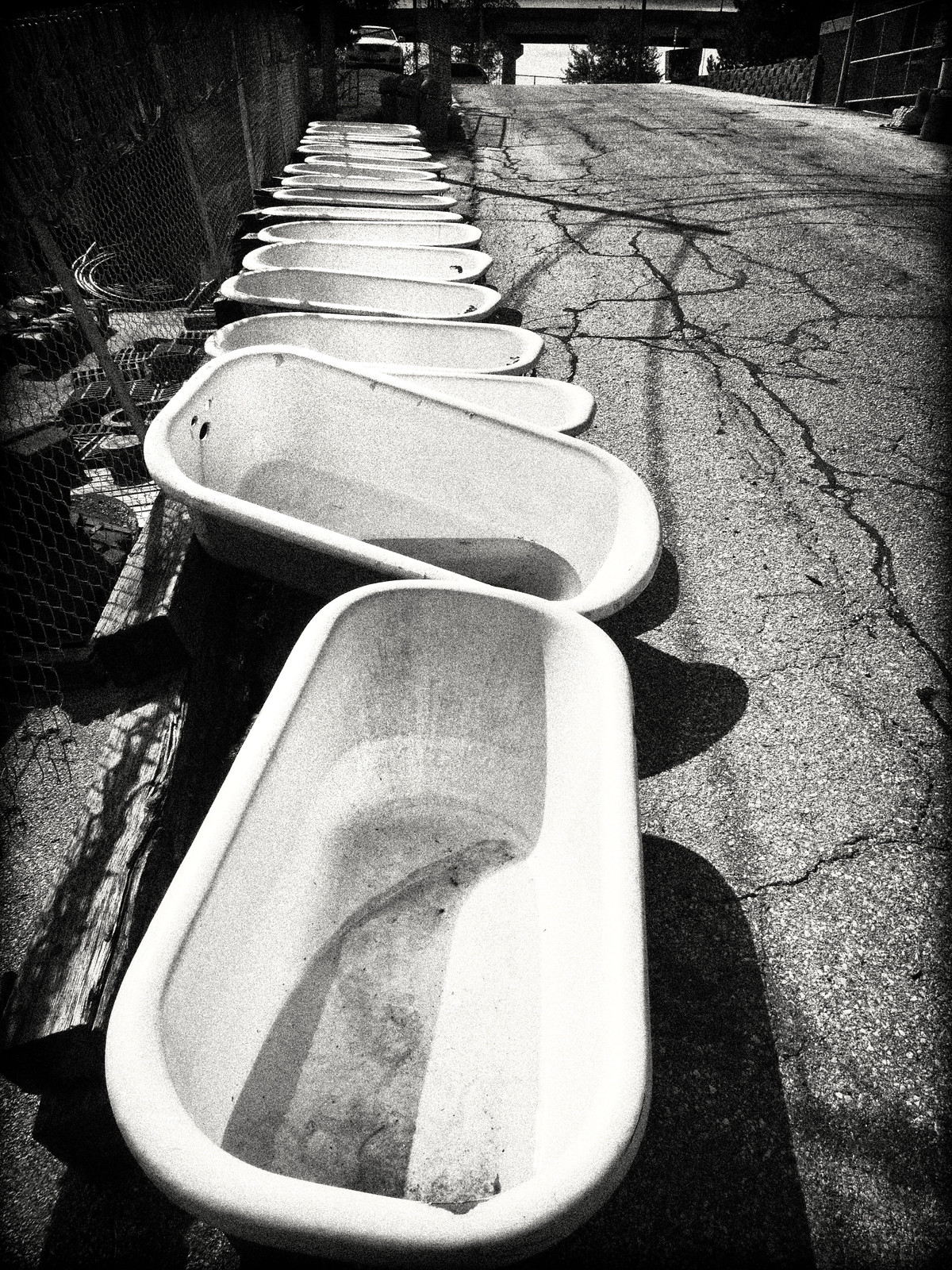The black-and-white photograph captures an intriguing outdoor scene on a cracked tarmac road. From the vantage point of the camera, the road extends away into the background, hinting at a potential journey. On the left side of the road, a series of approximately 15 to 20 discarded, white bathtubs form a single row stretching from the foreground into the distance. The bathtubs, which vary slightly in alignment, display a mix of orientations; the foreground bathtub shows its short end facing the viewer while subsequent bathtubs turn with their long sides facing the road. Some of these tubs appear to contain a liquid, adding to the scene's texture. The road itself is old, marked by numerous cracks visible especially on the right-hand side. Flanking the row of bathtubs is a chain-link fence that separates the street from an adjacent property. In the distance, the scene is completed by a parked car and the partial glimpse of a bridge, suggesting a blend of neglect and intentionality that could be aimed at artistic expression.